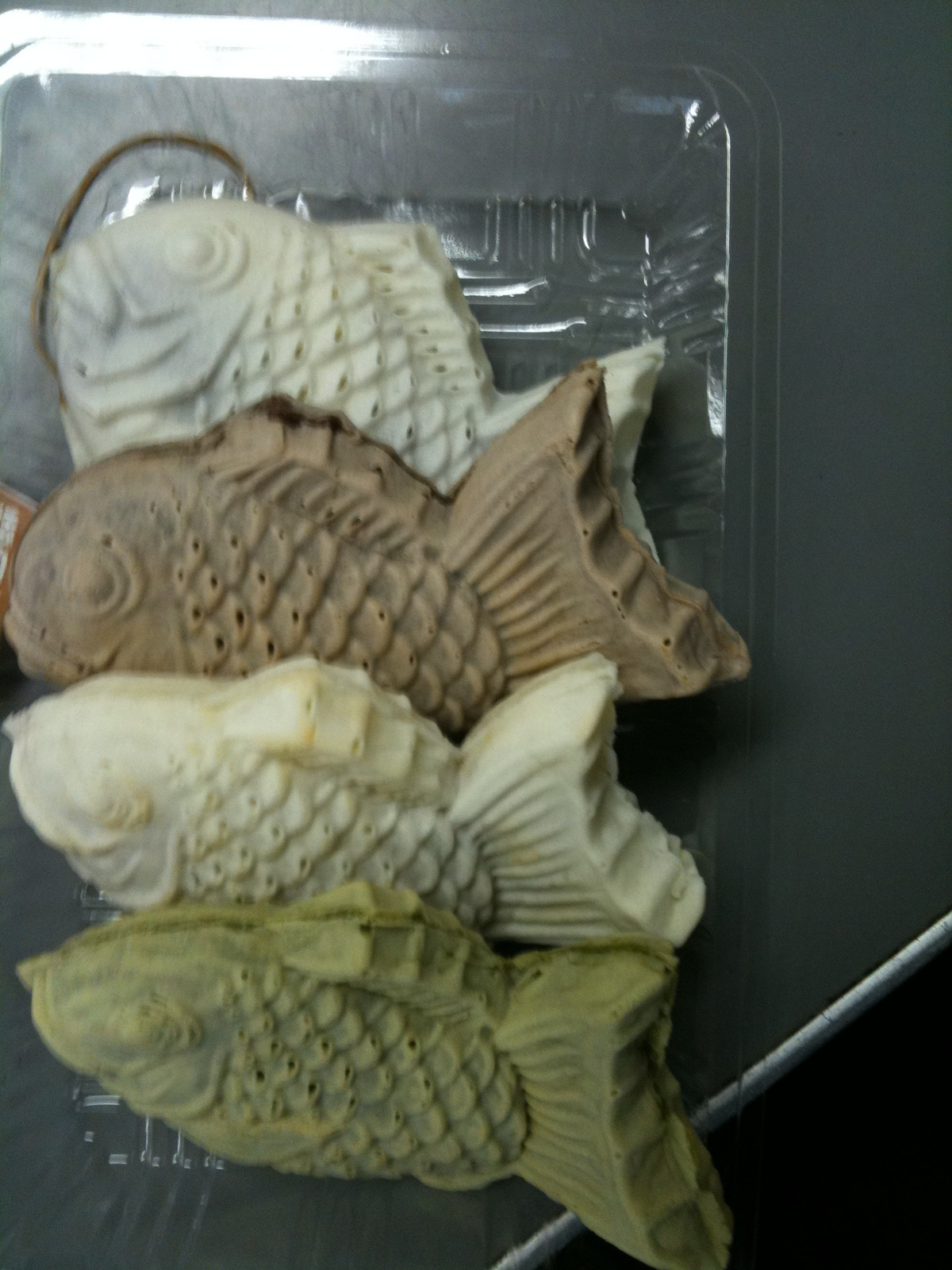The indoor photo, taken from above, captures a clear rectangular plastic container on a gray table with white edges. Inside the container are four fish-shaped cookies, each uniquely colored: the top one is white, followed by a brown one, then a cream-colored one, and finally a green one at the bottom. The cookies intricately feature details such as eyeballs, mouths, scales, fins, and tails. The brown fish has a piece of chocolate sticking out, tangibly touching the adjacent white fish, which is slightly tilted upwards. To the top left corner of the setting, a tan rubber band is visible. The plastic container appears to be a form tray, typically used for molding such intricately shaped cookies.